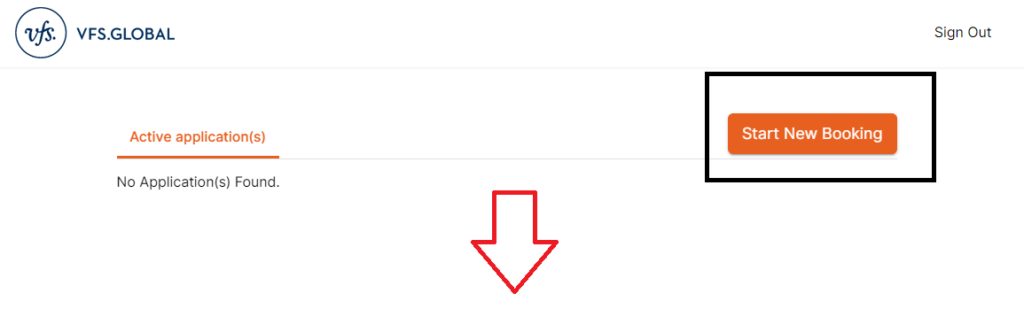On a white background, there is black text positioned in the upper left corner. To the right of a black circle with a white interior, the cursive initials "VFS" are inscribed. Adjacent to this, in uppercase regular text, it reads "VFS.GLOBAL." 

In the right-hand corner of the page, the words "Sign Out" are plainly displayed. Below this, nearer to the center-left, the text "Active Application(s)" appears in underlined orange letters. 

Towards the right-hand side, there is a black square containing a blue and orange button inscribed with "Start New Booking" in white text. Beneath the "Active Application(s)" section, the phrase "No applications found" is written in black.

Dominating the center of the page is a large red outlined arrow pointing straight downwards.

This information concludes the content of this page. Thank you to the team for their continued efforts, and it is noted that the completion award has increased to $3.35 per hour, likely reflecting the time required for these tasks.